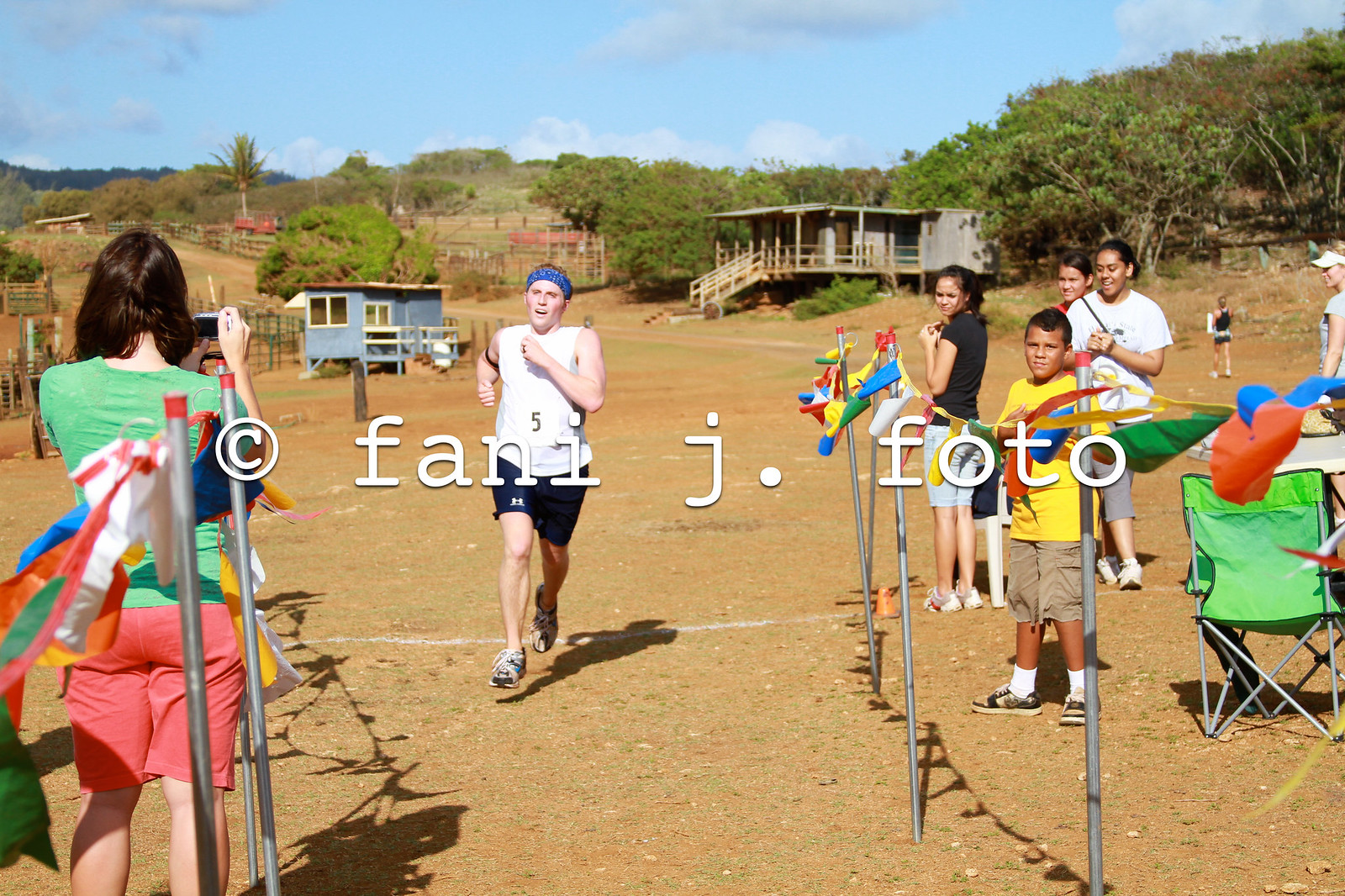The photograph captures an outdoor race event in a sandy, desert-like setting beneath a partially cloudy blue sky. The backdrop features verdant hills, scattered trees, and two small buildings—a light blue one resembling a chicken coop and a gray one with steps. Dominating the scene is a large wooden porch attached to a house. A runner wearing a white sleeveless shirt with the number five, blue shorts, running shoes, and a blue bandana around their head is prominently featured, sprinting towards a finish line marked by a white line in the dirt. Silver poles adorned with multicolored, hand-sized flags line the runway, vividly marking the race lane. Spectators, including several children and a woman in a green shirt and peach shorts, are actively engaged, some capturing the moment with their cameras. A green camping chair is positioned off to the side, adding to the casual atmosphere. The image is watermarked with "copyright Fanny J photo" in the center.